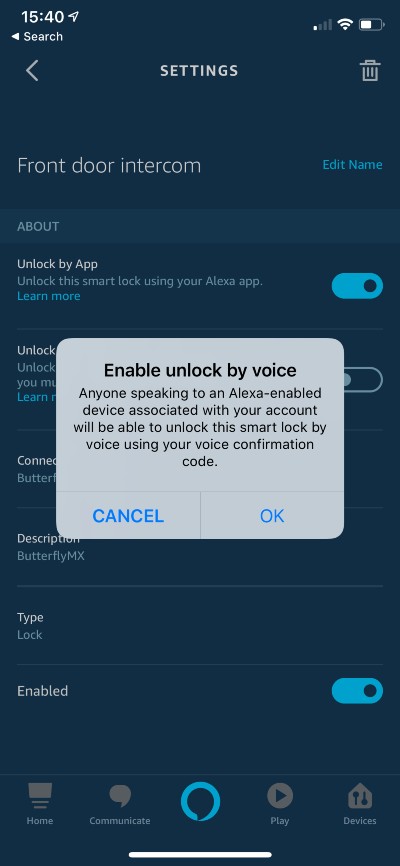Here is a refined and detailed caption for the provided image:

---

A screenshot of the Amazon Alexa app's settings page, featuring a dark blue background. At the top center, the word "Settings" is prominently displayed. To the left, an arrow icon points leftward, indicating a "back" function, while a trash can icon on the right suggests a delete option. Below, "Front Door Intercom" is displayed in large white font, with a smaller "Edit Name" link in blue font to its right.

Further down on the left side, the heading "About" is followed by the option "Unlock by App," accompanied by a toggle switch on the right that is turned on. Below that, "Unlock by Voice" is displayed, also with a toggle switch to the right, though this one is turned off.

In the center of the screen, a large white pop-up window appears, notifying the user to "Enable Unlock by Voice." The disclaimer below states that enabling this option will allow anyone speaking to the device associated with the account to unlock the smart lock by voice, using the user's voice confirmation code. The pop-up provides two options: "Cancel" on the left and "OK" on the right.

Below the pop-up, two additional settings categories are visible: "Type" and "Enabled." The "Enabled" category features a toggle switch that is turned on.

At the very bottom of the screen, a navigation bar includes five icons: a "Home" button, a "Communicate" button, a central blue Alexa button, a "Play" button, and a "Devices" icon on the far right.